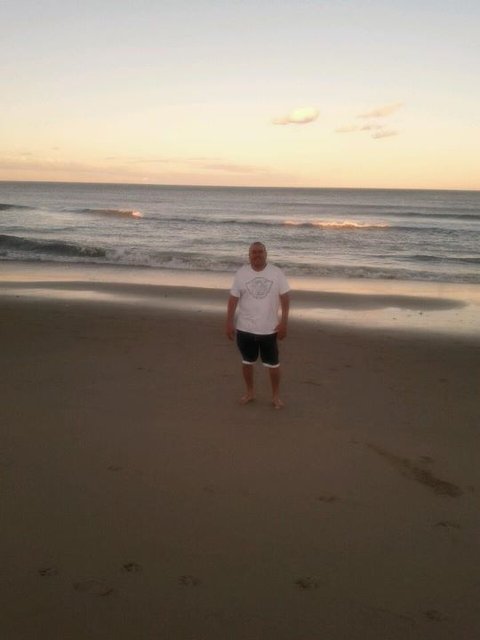The photo captures a serene beach scene, possibly around sunrise, with a vast stretch of brown sandy shore extending up to the tranquil ocean. The sky transitions from a soft yellow near the horizon to a clearer blue with a few scattered fluffy clouds, suggesting early morning light. Central to the image is a man standing barefoot on the damp sand, some distance from the gentle ripples of the sea. He is clad in black shorts featuring white stripes at the bottom and a white t-shirt with a gray insignia on the chest. Due to the image's low resolution and visible JPEG artifacts, finer details are indistinct, but his short dark hair and absence of accessories like hats or shoes are noticeable. The man is looking straight at the camera, appearing to smile faintly, with no one else present in this tranquil, solitary scene.